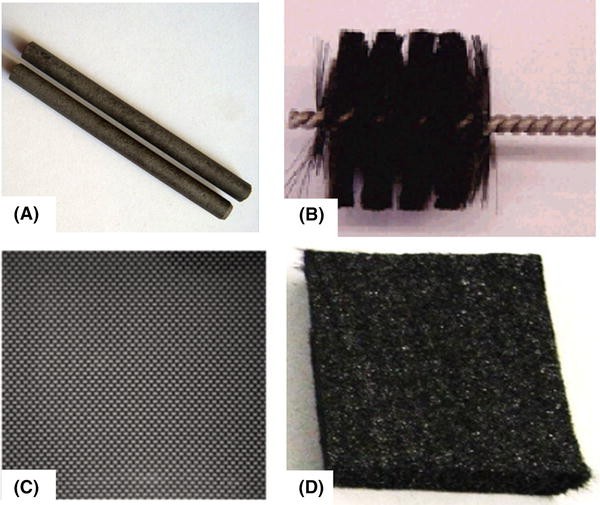The image consists of a collage of four individual photographs, each separated by white horizontal and vertical lines. Each section is labeled with an uppercase letter: A, B, C, and D, arranged in a grid format with A in the top left corner, B in the top right corner, C in the bottom left corner, and D in the bottom right corner.

- **A:** This image displays two dark gray metal bolts, prominently positioned against a contrasting background.
- **B:** This photograph features a helical tube with black bristles spiraling along its length, resembling a brush.
- **C:** The image showcases a piece of black mesh material, with its texture and structure clearly visible.
- **D:** This section depicts a black sponge-like material, which appears to be an umbrella pad. The pad is folded in half, and it is speckled with small white particles dispersed across its surface.

Each image is distinct, providing a detailed view of various materials and objects.